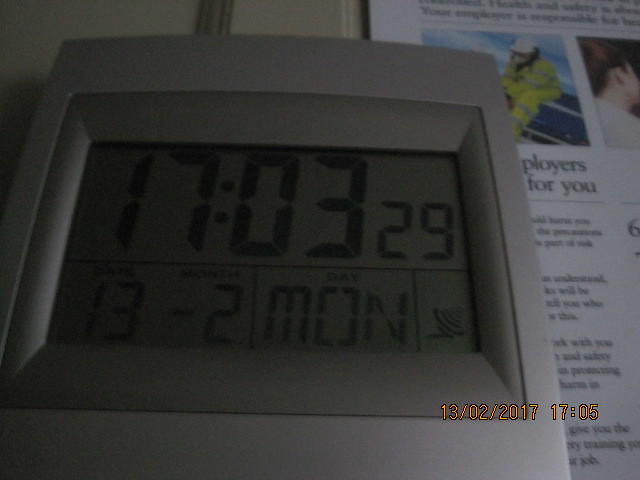This is an image of a digital clock displaying the time as 17:03:29. The date shown on the clock reads Monday, February 13. However, there is a discrepancy as the image timestamp indicates February 13, 2017, at 17:05. The photograph captures the clock's bright LED display against an unspecified background, contributing to a futuristic yet slightly anachronistic atmosphere due to the conflicting time details.